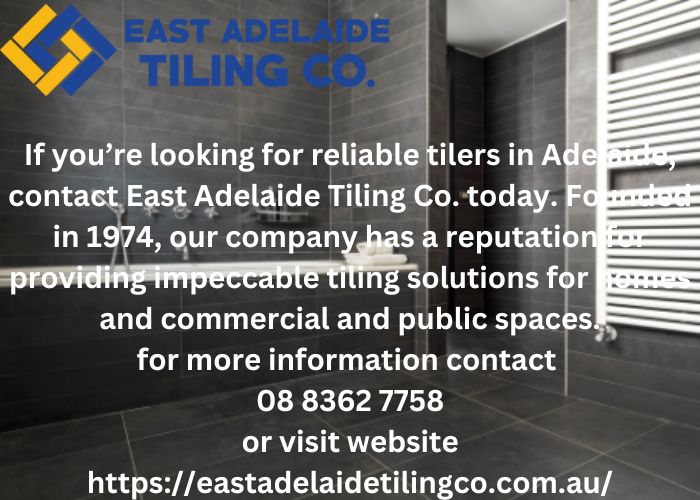The image features a promotional ad for East Adelaide Tiling Company, prominently displayed in the upper left corner in sky blue text. Adjacent to it, in the far left corner, is the company's blue and gold logo depicting two intertwined squares. The well-tiled background showcases a sleek, dark gray tiled shower, complete with visible faucets, a tile towel drying rack on the right side, and a soap holder, all extending up to the crown molding. Overlaying the image is white text that reads: "If you're looking for reliable tilers in Adelaide, contact East Adelaide Tiling Company today. Founded in 1974, our company has a reputation for providing impeccable tiling solutions for homes and commercial and public spaces. For more information, contact 08-8362-7758 or visit our website at https://eastadelaidetilingco.com.au." The combination of the detailed tiled shower and the informative text effectively highlights the company's professional tiling expertise.